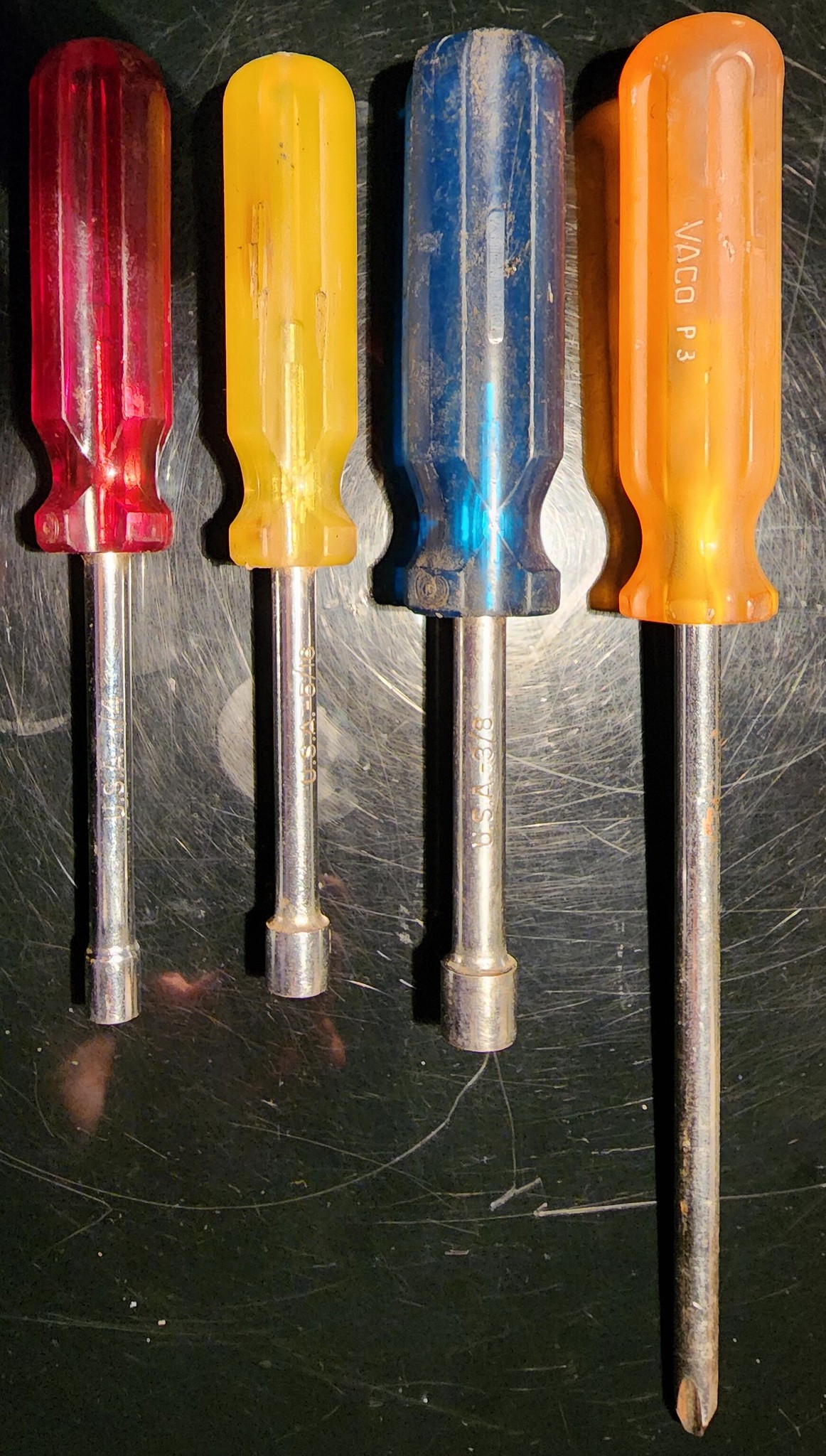This close-up photograph captures four screwdrivers laid out horizontally, covering the entire frame from left to right on a black metal surface that appears scuffed and scratched, indicative of frequent use, perhaps on a toolbox or within a drawer. The black background reflects light, adding a subtle shine to the scene. From left to right, the screwdrivers have handles in red, yellow, blue, and orange. The first three screwdrivers feature shorter stems with silver cylindrical ends designed for unscrewing bolts rather than standard screws or nails, identifying them as nut drivers. The red-handled nut driver is the first on the left, followed by the yellow and then the blue nut drivers. The final tool on the right, with an orange handle, is distinguishably longer and equipped with a pointed metal end, identifying it as a standard Phillips head screwdriver.